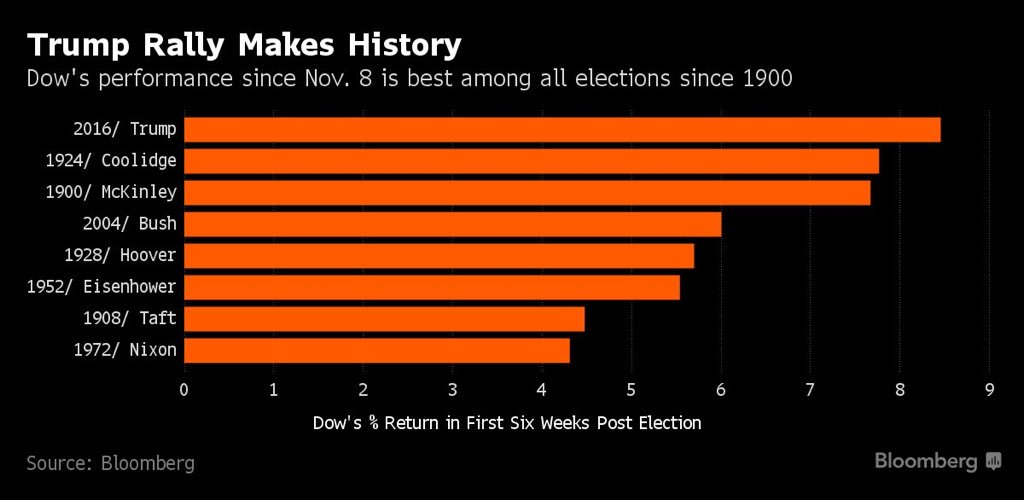A detailed line graph titled "Trump Rally Makes History" is displayed against a black background with white text highlighting the Dow's performance since November 8th. The graph compares the percent return of the Dow in the first six weeks post-election for various U.S. Presidents since 1900. 

The data points are represented by orange lines:
- **2016 - Trump:** Nearly reaching a 9% return.
- **1924 - Coolidge:** Approximately an 8% return.
- **1900 - McKinley:** Just below an 8% return.
- **2004 - Bush:** Around a 6% return.
- **1928 - Hoover:** Close to a 5.5% return.
- **1952 - Eisenhower:** Slightly under a 5.5% return.
- **1908 - Taft:** About a 4.5% return.
- **1972 - Nixon:** Slightly over a 4% return.

The source of the information is credited to Bloomberg, with the Bloomberg logo also appearing on the right side of the image. The caption emphasizes the exceptional market performance following Trump's election, positioning it as the highest since 1900.